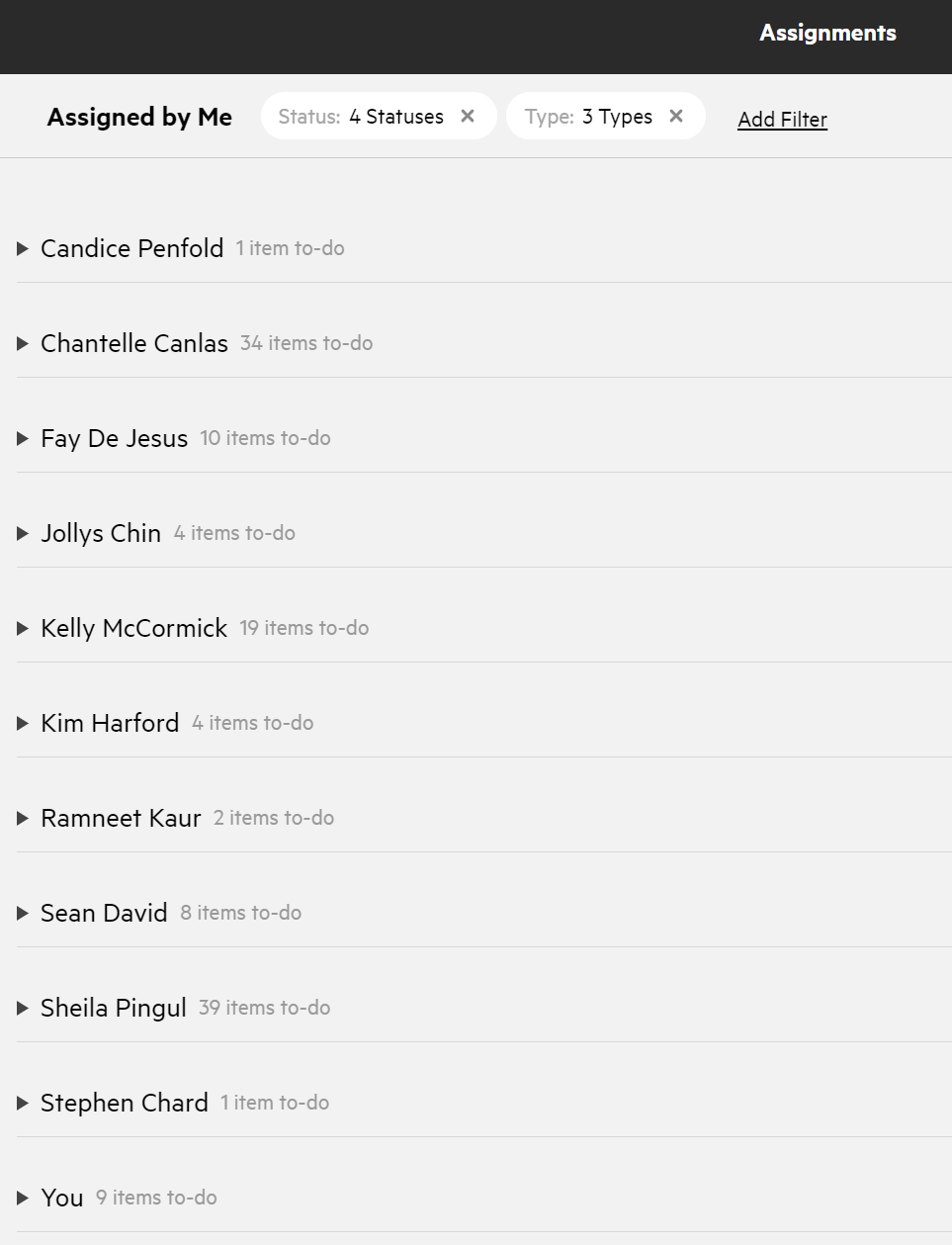**Screenshot of To-Do App Interface: Comprehensive Task Overview**

The screenshot displays a to-do application interface, predominantly featuring a black banner at the top with the word "Assignments" in white letters. Below the banner, the interface is organized into several columns labeled from left to right: "Assigned by Me," "Status" (with four different statuses), "Type" (listing three types), and "Add Filter."

The task list section details assignments allocated to various individuals, each row starting with a person's name in bold black text next to a symbol resembling a black play button. The to-do items attributed to each person are listed in gray text. The detailed breakdown of tasks assigned to each individual is as follows:

- **Candice Penfold**: 1 item to do
- **Chantel Canlis**: 34 items to do
- **Faye de Jesus**: 10 items to do
- **Jolly's Chin**: 4 items to do
- **Kelly McCormick**: 19 items to do
- **Kim Harford**: 4 items to do
- **Remnit Karr**: 2 items to do
- **Sean David**: 8 items to do
- **Sheila Pingle**: 39 items to do
- **Stephan Charr**: 1 item to do
- **You**: 9 items to do

Each name is followed by the corresponding number of tasks, providing a clear and organized overview of assignments within the application.